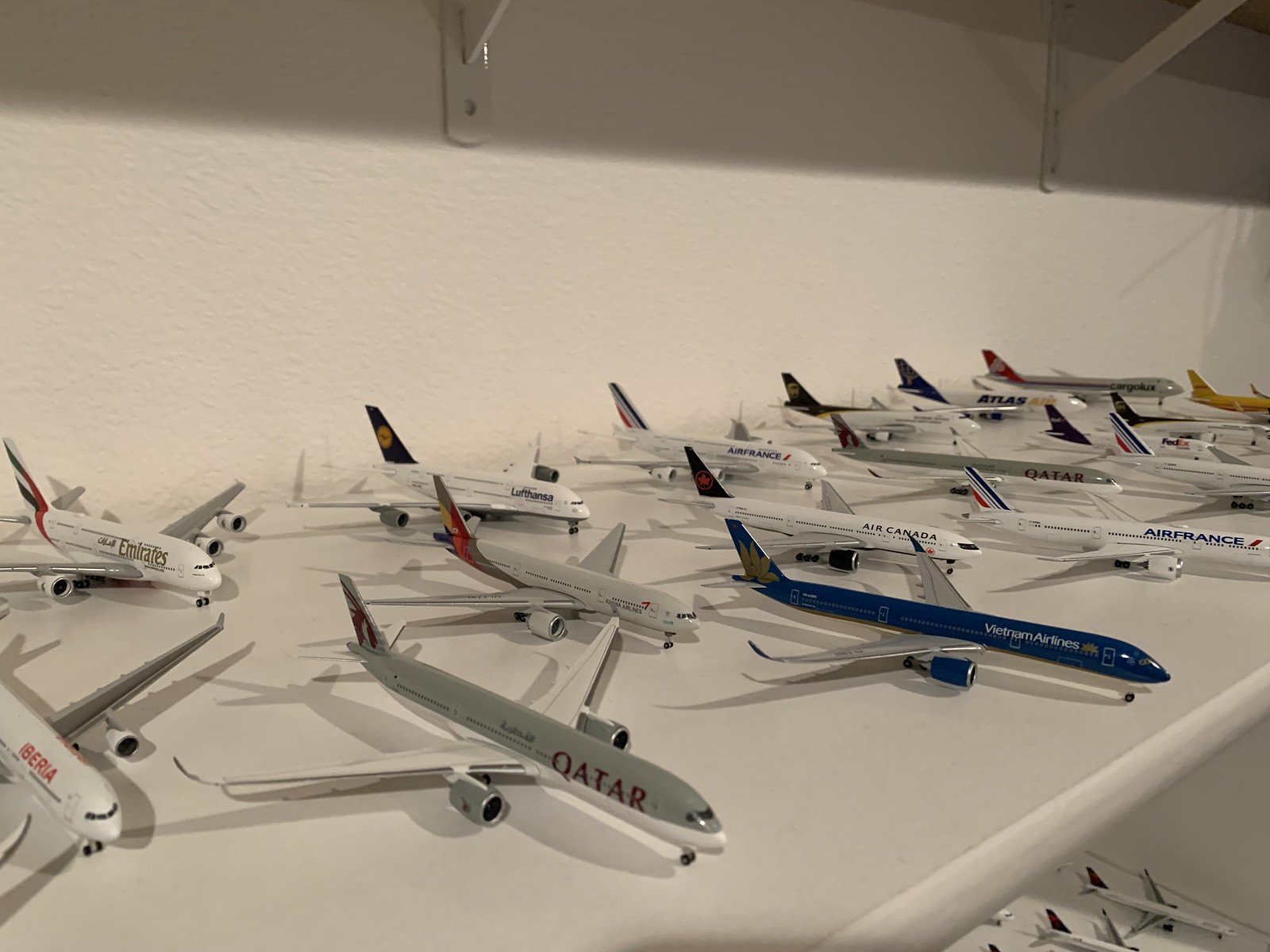This indoor color photograph showcases a meticulously arranged collection of approximately 20 detailed model airliners displayed on a pristine white shelf against a white wall. Each model is uniformly oriented with its tail to the left and nose to the right, enhancing the display's orderly appearance. The liveries of various international airlines adorn the models, including Qantas, Emirates, Iberia, Qatar, Air France, Air Canada, Virgin Atlantic, Vietnam Airlines, Lufthansa, FedEx, and Atlas. In the foreground, the precise detailing of the liveries is crisp and clear, with notable models like the Airbus A380 in Emirates colors and a Boeing 767 in Qantas colors standing out. The background models are slightly out of focus, adding a sense of depth to the image. The photograph also captures a glimpse of another shelf below, also populated with model airplanes, as well as the brackets supporting the upper shelf. Various hues like blue, gray, and yellow among the predominantly white-bodied models add to the visual interest of the orderly display.